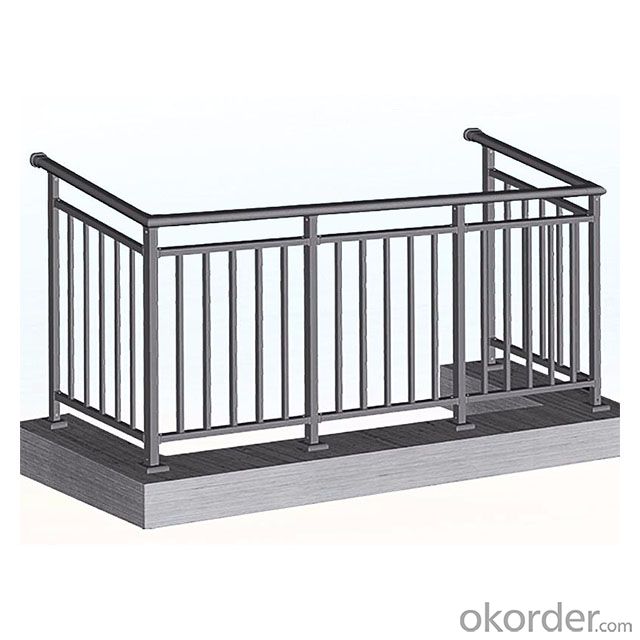The image is a computer-generated digital drawing depicting a rectangular metal railing, potentially intended for an apartment balcony. The railing, which appears to be approximately 3 feet in depth and 9 feet across, stands on a wood-grained base rendered in shades of gray, matching the overall gray color palette of the entire structure. The railing itself is 3 to 4 feet high and features vertical bars supported by horizontal metallic frames, with each panel containing five bars. There are three panels along the front and one on each side. The product is showcased on an Infinite White background with the text "OKOrder.com" in gray font located in the bottom right corner, indicating the fencing is available for purchase on the mentioned website.